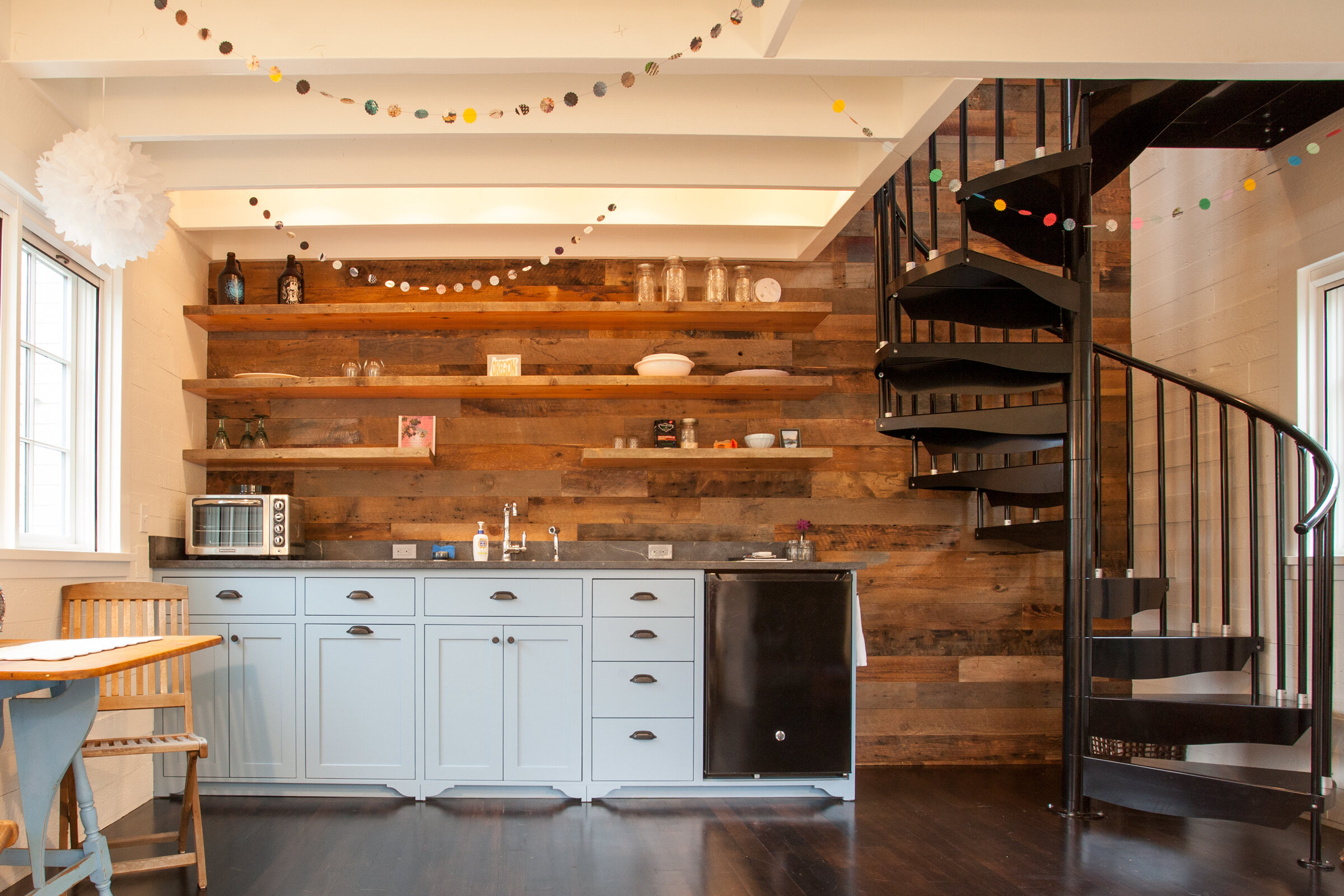This detailed color photograph captures a stylish, open-concept kitchen with striking modern elements. The lower cabinetry consists of three white, wood-finished vanity sets with brown handles. On the right-hand side, a dishwasher with a sleek, black-silver finish is integrated into the cabinetry, while the left-hand side features a silver chrome toaster oven. The central vanity accommodates a kitchen faucet and spray handle, presumably indicating the sink's location. 

Above the counter, the wall is adorned with horizontal, multi-colored wooden planks and is accented with three wooden shelves holding an assortment of bowls, plastic containers, seasoning bottles, and syrup bottles. The shelves add both functionality and ornamental charm to the space. The floor is a polished, dark wood that reflects the cabinetry, enhancing the room's aesthetic.

The wall on the left hosts large windows that invite natural light, complemented by a small dining table paired with two pale wooden chairs. Flanking the right side is a captivating black spiral staircase with an aluminum chrome finish, ascending from the hardwood floor and decorated with small tea candles on each step. The right-hand wall is clad in white brick, adding a textured contrast.

The ceiling features exposed beams adorned with strings of decorative balls, reminiscent of celebratory festoons or party lights, alongside a modern Ikea-style light fixture resembling a white plastic puff. The combination of these elements creates a cozy yet contemporary atmosphere that is both functional and inviting.